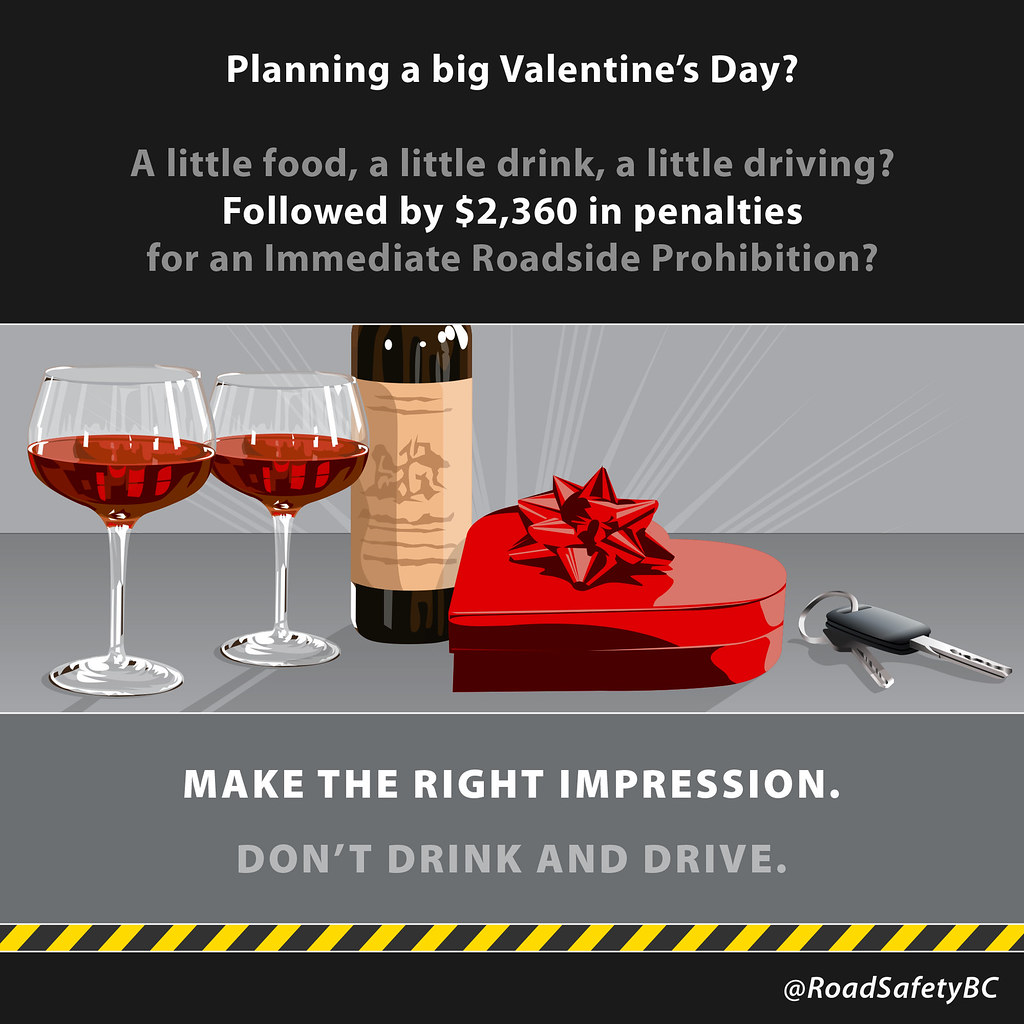The advertisement is designed to resemble a Valentine's Day card and serves as a public service announcement against drinking and driving. The top portion of the card features a black background with bold white text asking, "Planning a big Valentine's Day?" A secondary question in smaller gray text follows: "A little food, a little drink, a little driving?" Below this, in white text, it ominously states, "followed by $2,360 in penalties", with a gray question underneath reading, "for an immediate roadside prohibition?"

Transitioning to the middle section of the card, the background shifts to a light gray at the top and a darker gray at the bottom, mimicking a wall and countertop setting. The focal point comprises an illustration of two wine glasses filled with red wine positioned to the left of a wine bottle. Beside the wine bottle, a heart-shaped gift box adorned with a red bow signifies a Valentine's Day gift. To the far right of the box, a set of car keys lies prominently, reinforcing the theme.

Below this imagery, a line runs across the card, separating it from a message in white text, "Make the right impression". This message is followed by the cautionary advice in gray text, "Don't drink and drive." The bottom edge of the card features a diagonal pattern made up of gray and yellow stripes, akin to caution tape. Finally, a black border at the bottom right corner displays the text "@roadsafetyBC" in white, anchoring the ad to its source.